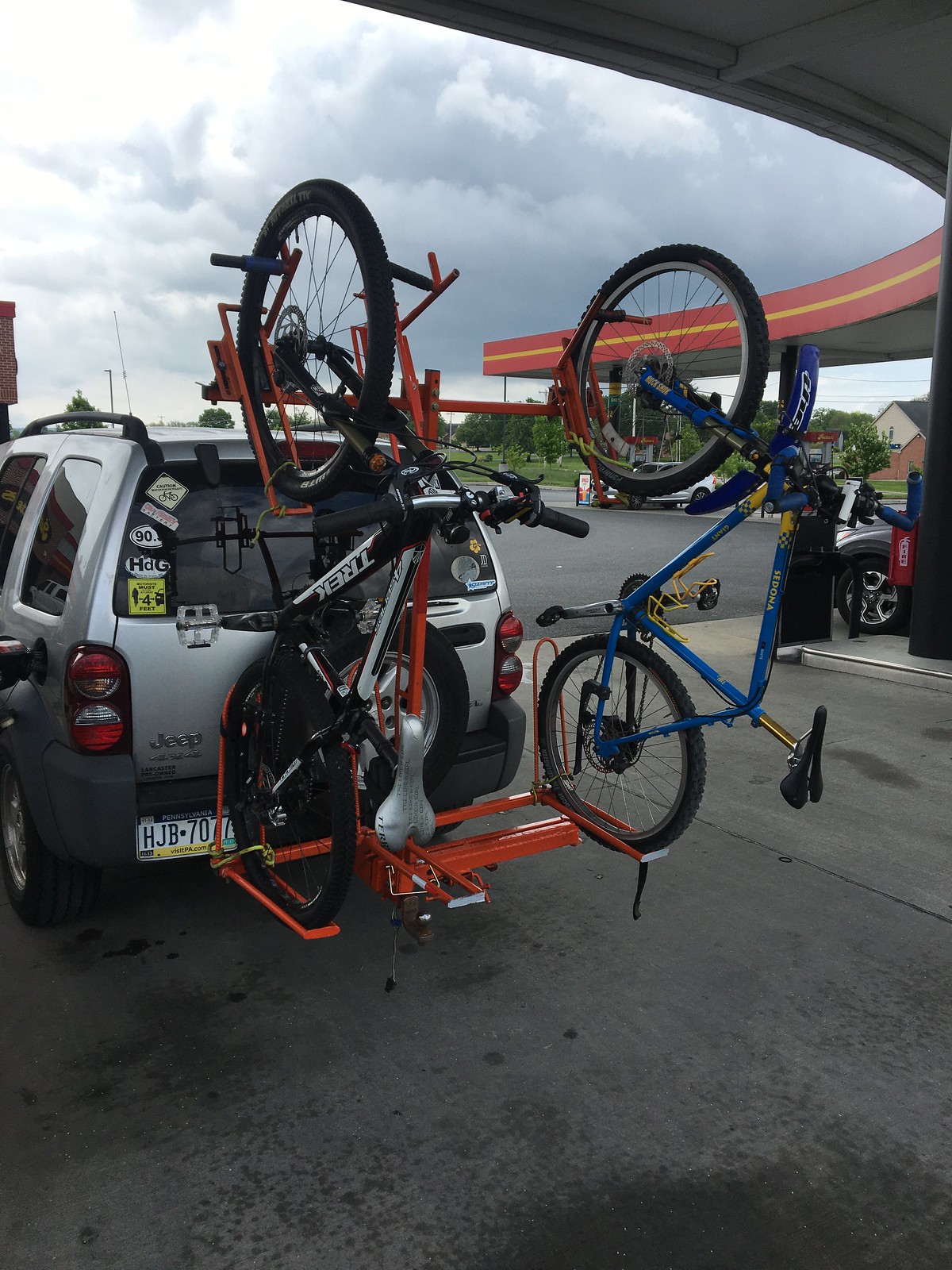The photograph features a compact silver station wagon, possibly a small SUV, located centrally in the frame towards the left side, as it departs a gas station. The vehicle, equipped with black roof racks and a European license plate, supports an orange metal bike rack on its rear. This bike rack hoists two bicycles vertically, with their front wheels elevated into the air. The bicycle on the right is blue and black, while the one on the left is red and black. The vehicle is parked on a gray cement surface, and two fuel pumps along with the awning above them are visible to the right. The awning is notable for its red color accented by a yellow stripe. In the far background, you can see the outline of trees and the edge of a house. Above, the sky is predominantly gray with a mixture of white clouds, presenting a somewhat overcast appearance.